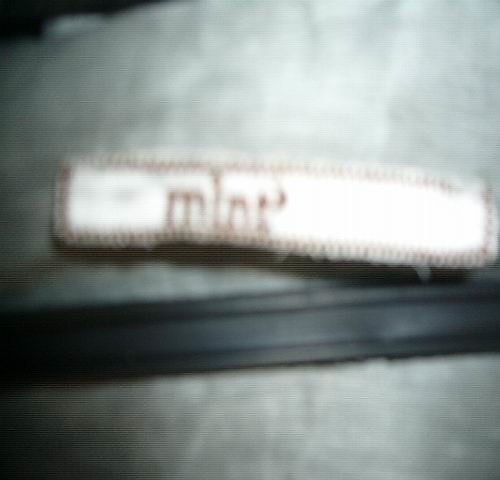An extremely blurry and out-of-focus image depicts a scene that is difficult to decipher. The background consists of a mix of gray and white hues, creating a visually ambiguous backdrop. At the bottom of the image, a vertical stripe can be observed, bordered by two black raised lines on each side. Above this stripe lies a white rectangle, potentially adorned with brown stitching around its edges. Inside this white rectangle, there is some text that remains too blurred to clearly identify. The text appears to form a four-letter word, but its precise language and meaning are indeterminate.